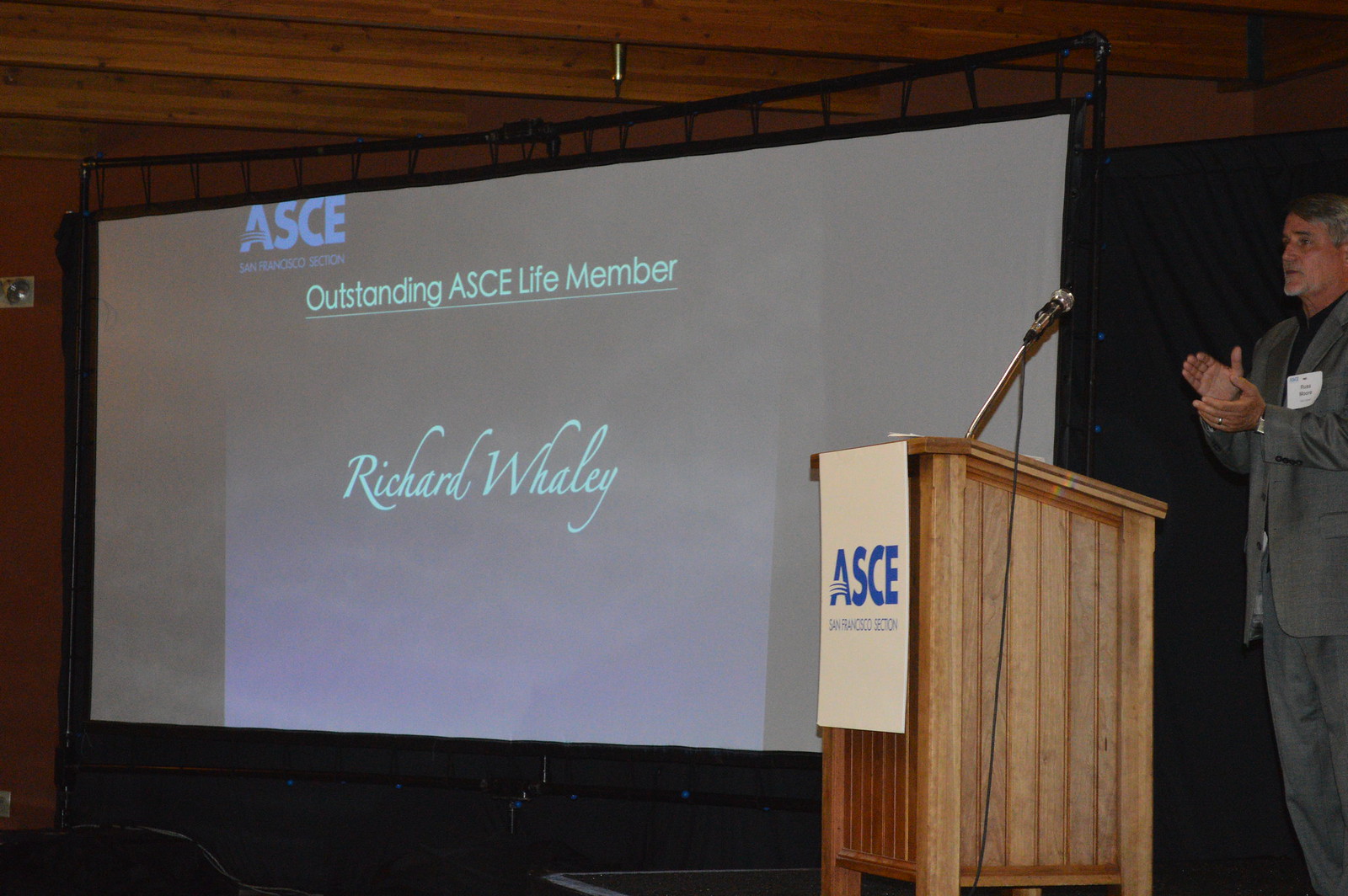The image appears to be taken indoors, possibly at a hall or convention. Dominating the left and center of the picture is a large projection screen, surrounded by a black fabric backdrop. On the screen, in blue letters, it reads "ASCE," followed by "Outstanding ASCE Life Member," and the name "Richard Whaley." To the right of the screen is a wooden podium with a banner displaying "ASCE" in blue lettering on a cream background. A man in an olive-gray suit, wearing a name tag on his left breast and sporting dark hair with a slight gray beard, stands behind the podium. The man is mid-applause, indicating that he might be celebrating or announcing the accolade for Richard Whaley. The ceiling features wooden slats running from left to right, adding a rustic character to the room.